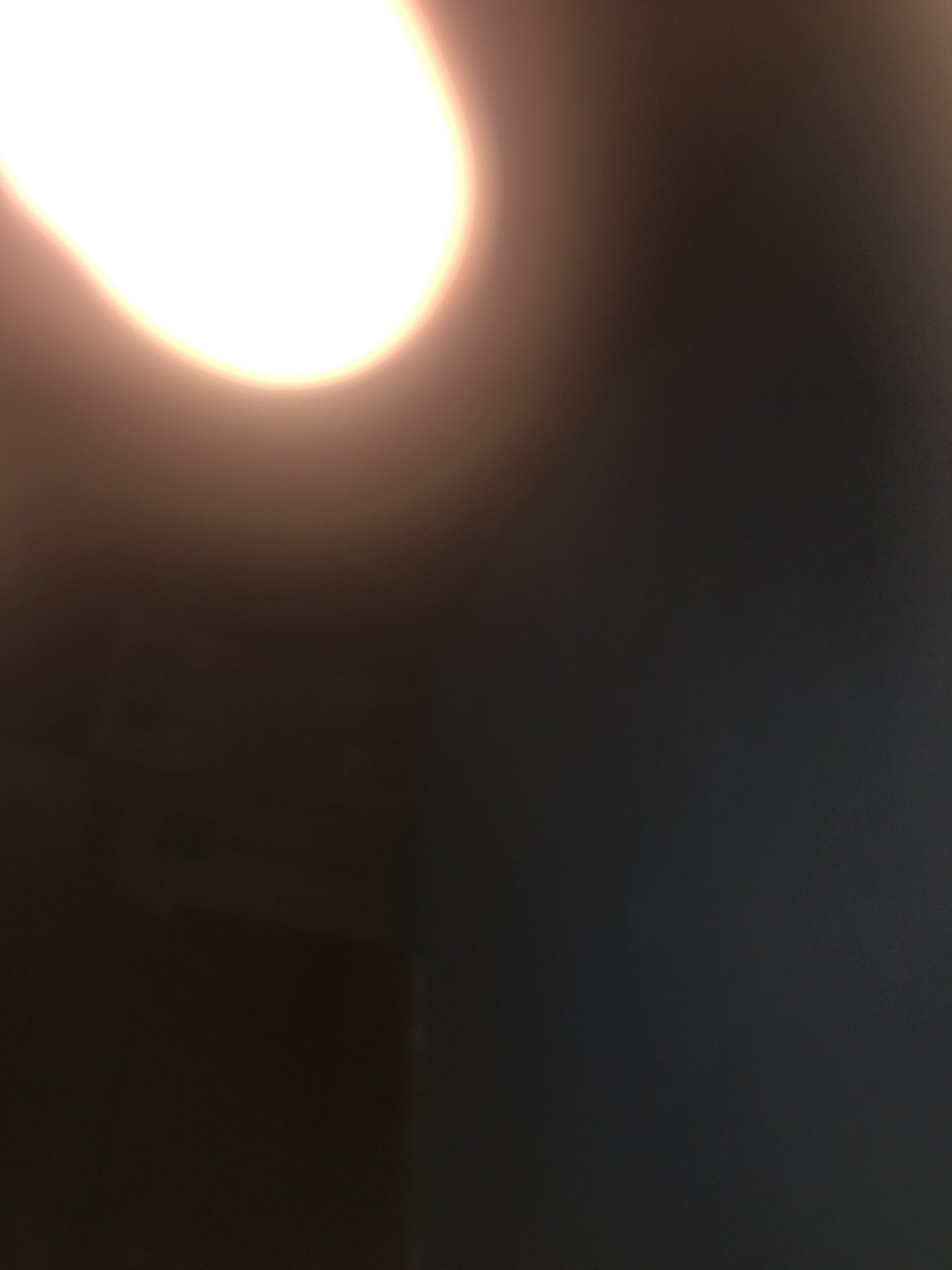The photograph depicts a dim, dark-colored room with blurred details and differing shades of darkness. The background consists of a dark blue to gray wall, with predominantly black areas on the left, right, and top sides. The far-right side also features an ironing board-shaped object, leaning against boxes on a shelf. The shelf itself is brown with yellow or white boxes on its top, including what might be a toolbox with two black clamps on it, though details are obscured.

Dominating the upper left corner of the image is a very bright yellow light with an orange outline and a U-shaped glow around it, radiating an orangish hue. This intense light blows out much of the photo, making the surrounding features difficult to discern. The overall image is close-up and out-of-focus, likely taken from ground level looking up, with substantial blurring that adds to the difficulty in identifying more specific elements within the room.